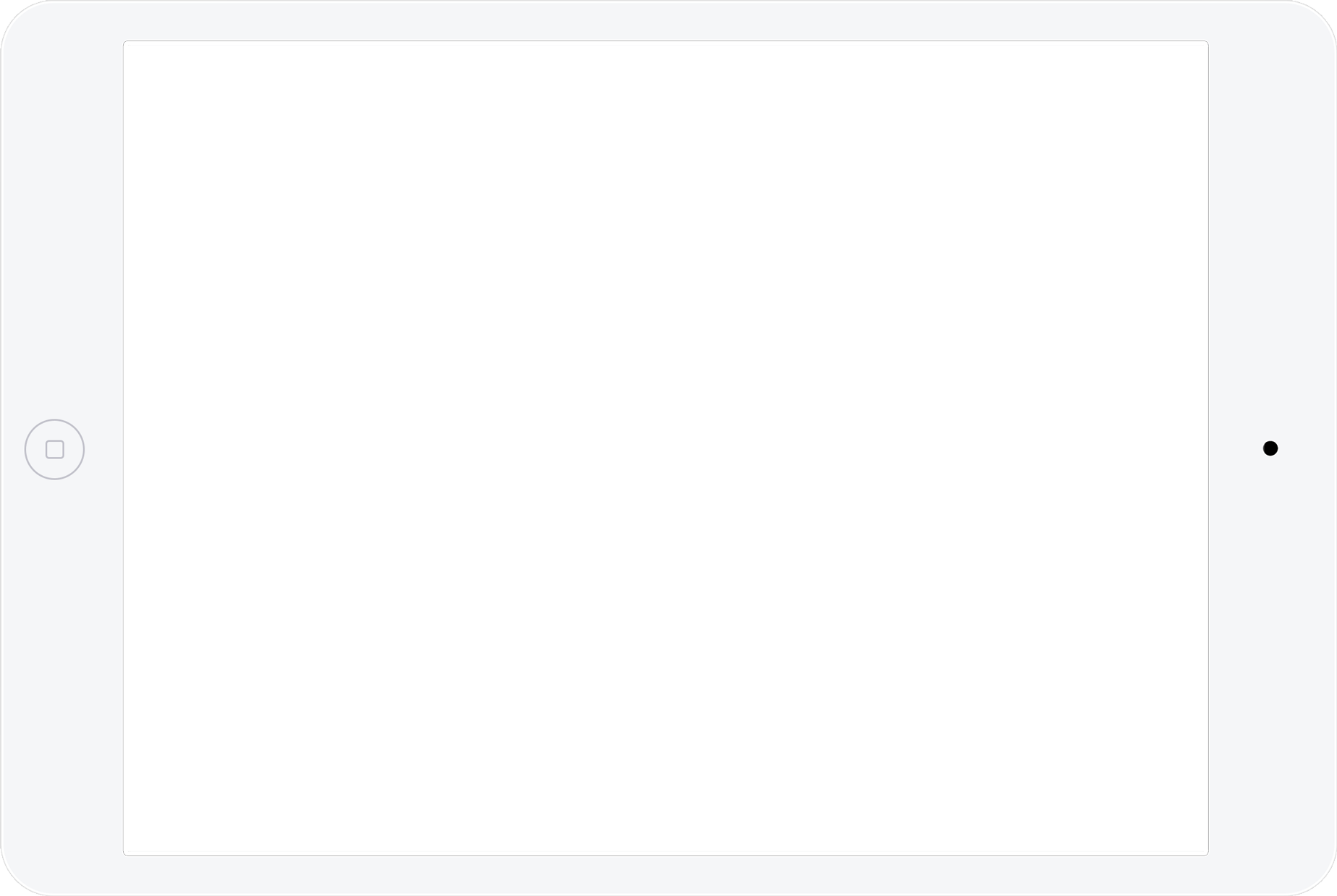The image depicts a predominantly blank screen encased in a border. The border along the top and bottom edges is thin and gray, while the left and right edges are notably thicker. Positioned midway down the left border, there is a circle containing a square, which appears to resemble an on/off button. In contrast, centered on the right border, there is a small black dot with no clear indication of its purpose. The main portion of the screen within the border is entirely white and devoid of any additional elements or markings.